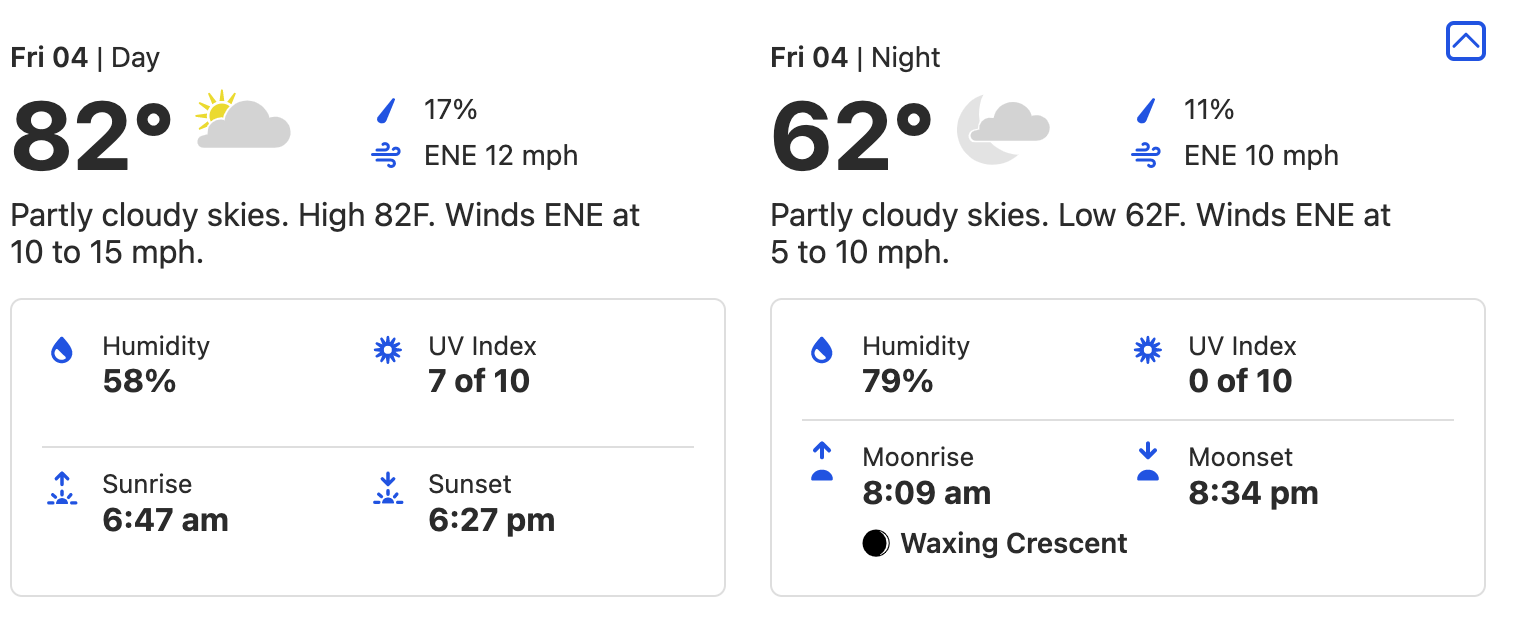The image depicts a detailed weather forecast for Friday, presented in two sections side-by-side against a white background. 

**Left Section: Friday Daytime Forecast**
- **Date and Day:** Friday, April 4th.
- **Temperature:** High of 82°F.
- **Weather:** Partly sunny with partly cloudy skies.
- **Winds:** Northeasterly at 10 to 15 mph (commonly 12 mph).
- **Chance of Rain:** 17%.
- **Humidity:** 58%.
- **UV Index:** 7 out of 10.
- **Sunrise:** 6:47 AM.
- **Sunset:** 6:27 PM.
- **Visual Elements:** There are text boxes in gray around humidity, UV index, sunrise, and sunset, as well as dividing lines between these elements.

**Right Section: Friday Night Forecast**
- **Temperature:** Low of 62°F.
- **Weather:** Partly cloudy skies.
- **Winds:** East-northeast at 5 to 10 mph.
- **Chance of Rain:** 11%.
- **Humidity:** 79%.
- **UV Index:** 0 out of 10.
- **Moonrise:** 8:09 AM.
- **Moonset:** 8:34 PM.
- **Moon Phase:** Waxing crescent.
- **Visual Elements:** Similar to the daytime forecast, this section also has gray text boxes around humidity, UV index, moonrise, and moonset, with lines separating these categories.

**Color Scheme:** The image primarily uses white, black, yellow, gray, and blue for its text and graphic accents.

**Additional Notes:** The forecast information is sectioned off with gray rectangles and dividing lines for clarity between different weather metrics.